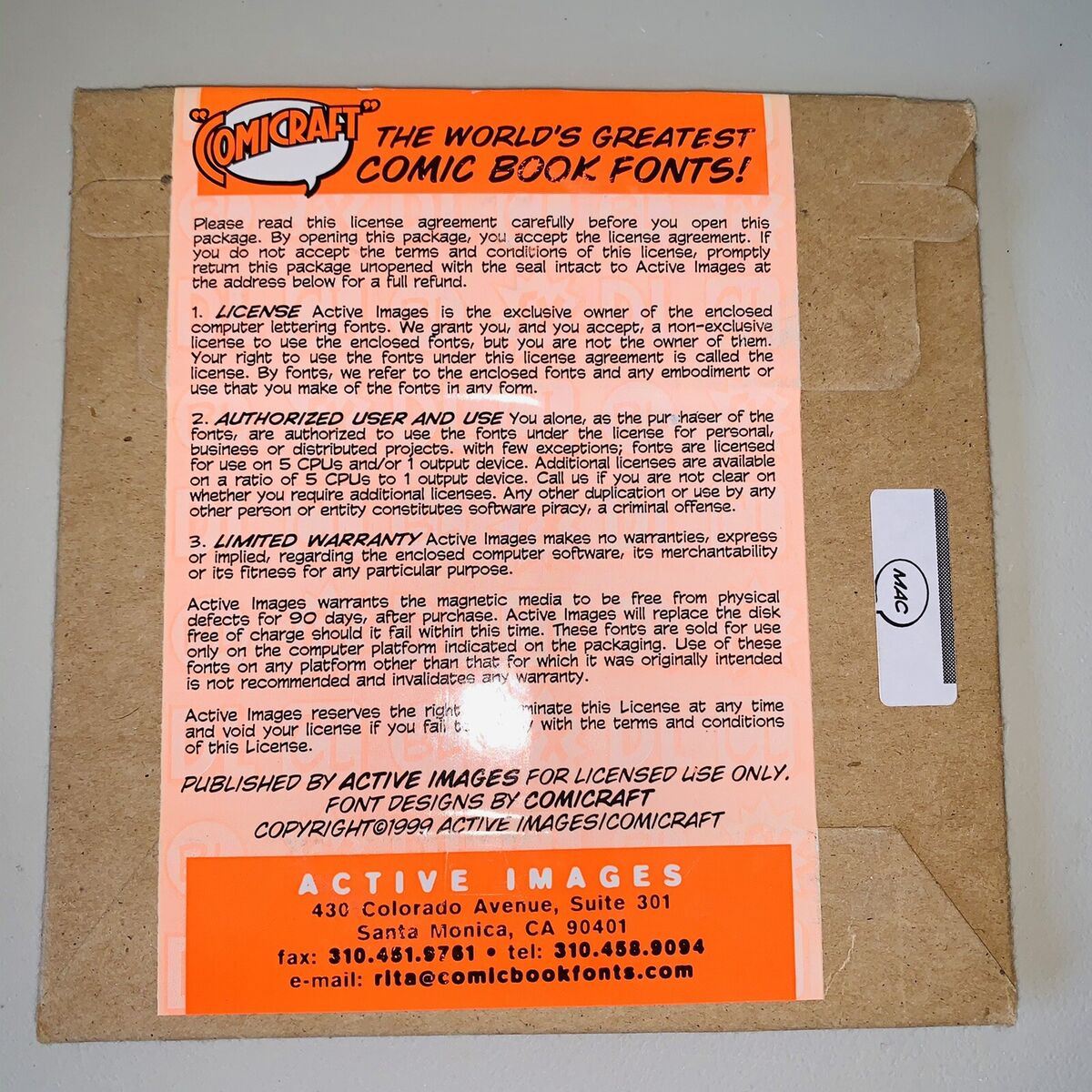The image shows a large brown mailing envelope placed atop a cardboard box labeled "MAC" on the right side, adorned with a distinctive orange label. The label, split into a bright orange top and bottom with a light pinkish-salmon middle, features a speech bubble at the top stating “Comicraft, the world’s greatest comic book fonts.” Beneath the title, the envelope contains a detailed licensing agreement in black font. This agreement outlines the terms and conditions for using Comicraft's fonts, including provisions for licensing, authorized users, use limitations, and a limited warranty. The bottom of the label bears a statement that says "Published by Active Images for licensed use only. Font designs by Comicraft," accompanied by copyright information from 1999. It also provides contact details for Active Images: an address at 430 Colorado Avenue Suite 301, Santa Monica, CA 90410, a fax number (310-451-9761), a telephone number (310-458-9094), and an email (Rita at comicbookfonts.com).